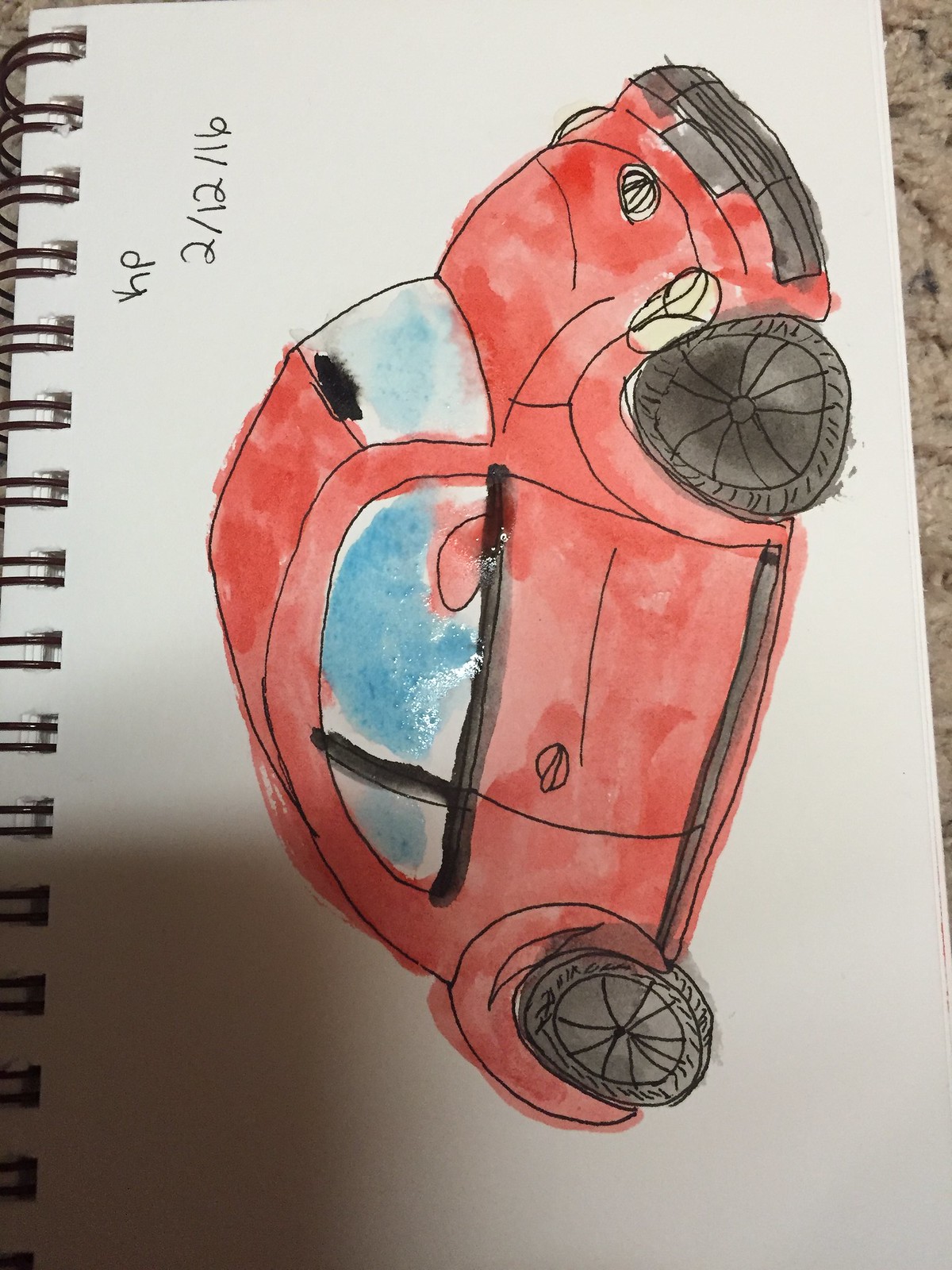A detailed pencil sketch of a classic red Volkswagen Beetle is depicted on a vertically-oriented page. The Beetle, with its signature curved body and black standard tires, is meticulously drawn, emphasizing both its charm and simplicity. The entire sketch is rendered in pencil, showcasing a draft-like quality with visible strokes. This artistic piece is set against a clean, white binder. To the upper right-hand corner, the artist's initials, "KP," along with the date "2-12-16," are inscribed, adding a personal touch and a timestamp to the artwork. The Beetle faces upwards on the page, seemingly ready for an adventurous drive.